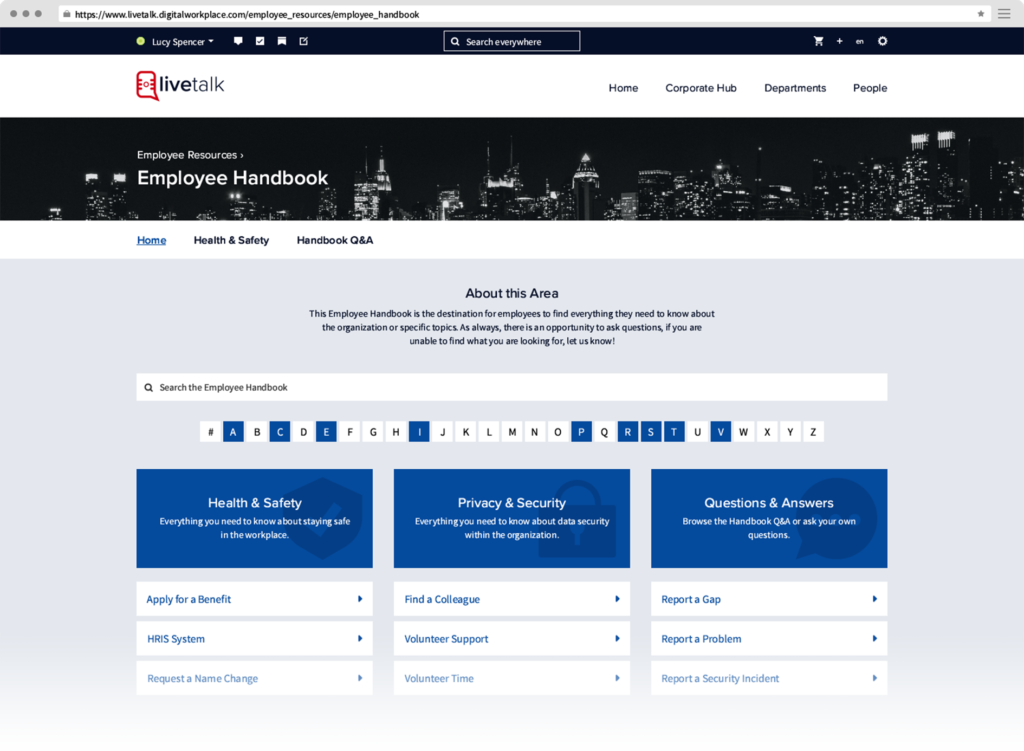The photo captures an open laptop showcasing a website titled 'Live Talk,' identifiable by its distinct red microphone logo positioned at the top. The website's user interface features multiple menus, including Home, Corporate, Hub, Departments, and People. Situated above these menus is a search bar labeled 'Search Everywhere,' accompanied by a shopping cart icon. On the top left side, the username 'Lucy Spencer' is displayed, alongside several icons for messages (speech bubble icon), note-taking, a ribbon, and a check mark.

The central content of the screen is focused on a section labeled 'Employee Handbook,' which falls under the broader category of 'Employee Resources.' Within this section, there are three sub-menus: Home, Health & Safety, and Handbook Q&A, with the current selection being the Home tab. The introductory text in this area explains that the Employee Handbook serves as a comprehensive resource for employees, providing essential information about the organisation and various specific topics. It highlights the option for employees to ask questions if they can't find the information they need.

Below this explanatory text, there is another search bar specifically for navigating the Employee Handbook. Various topics are listed from A to Z, with suggestions for quick access. Examples of these topics include 'Apply for Benefits,' dividing further into three main sections: Health & Safety, Privacy & Security, and Questions & Answers. Each of these sections features detailed subtopics to facilitate easy navigation and information retrieval.